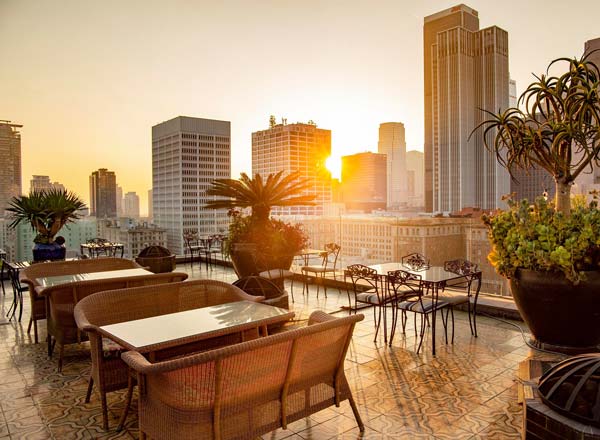A stunning rooftop setting in a large city, adorned with a variety of seating arrangements for visitors to relax and enjoy the view. The scene is illuminated by the sunset casting warm hues between tall skyscrapers and smaller buildings. The terracotta tiled floor adds to the ambiance, complementing the wrought iron seats and tables, along with glass tables outfitted with cushioned metal chairs. Large potted plants, some featuring pine trees surrounded by vibrant geraniums, and cedars around wicker-style tables, contribute to the lush greenery of the space. Though currently unoccupied, the rooftop exudes an inviting, upscale atmosphere perfect for dining, with a fan spinning as part of the air conditioning system, indicating a nearby restaurant or bar.